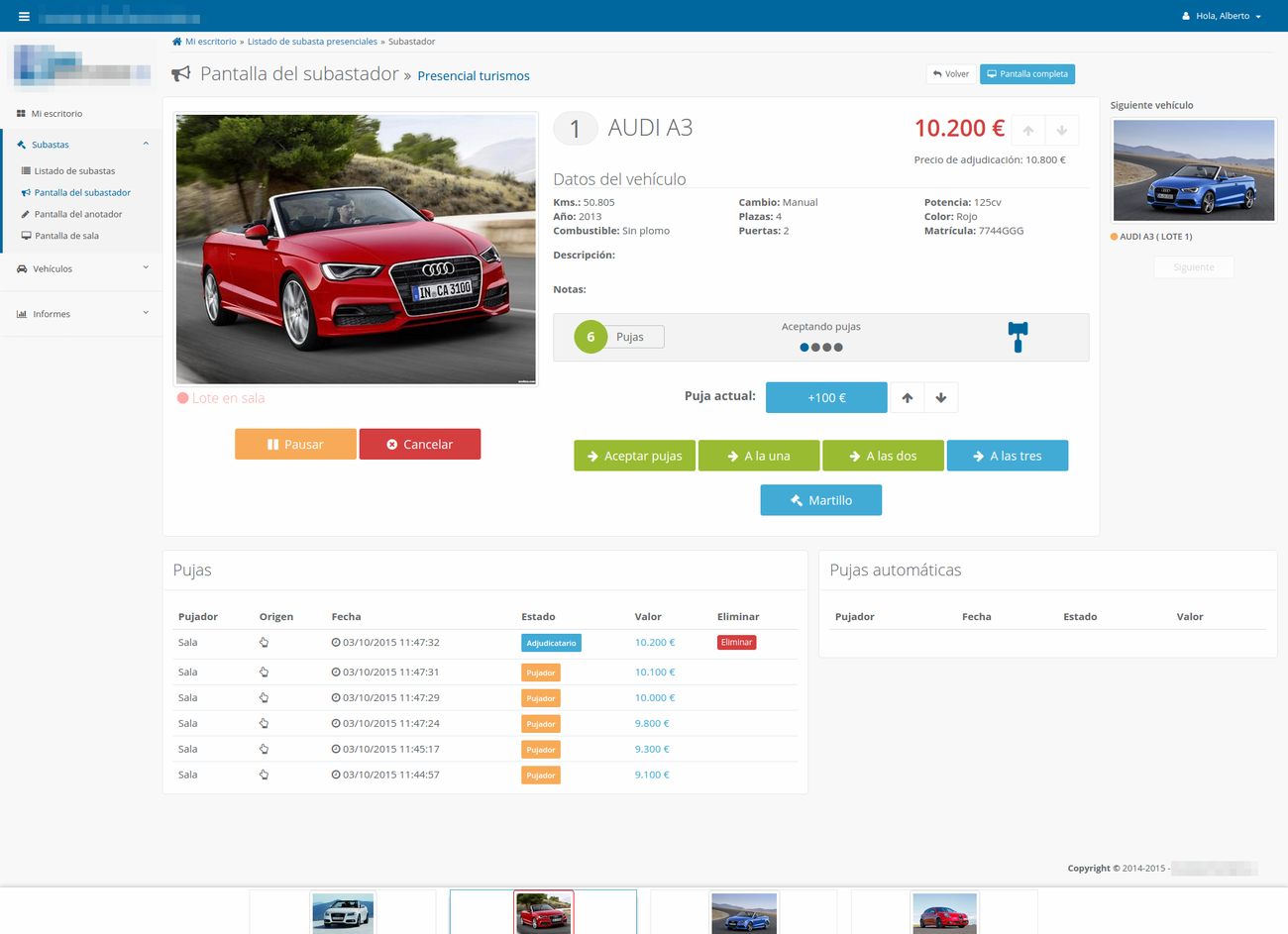The image depicts a detailed Spanish-language web page specializing in the resale of cars, specifically featuring the Audi A3. Prominently, in the upper left corner, there is a striking red convertible Audi A3 driving along a deserted road with trees and sandy terrain in the background. The accompanying price is listed as 10,200 Euros, indicating it is likely a second-hand vehicle. To the right of this main image, there is a smaller picture showcasing a blue convertible version of the Audi A3. The lower portion of the page contains various colored boxes—orange, red, green, and blue—each presenting different details and prices associated with the vehicles. Amid the complexity of the page are numerous links, buttons, and possibly auction elements where users can place bids, all aimed at facilitating the sale or trade of cars.